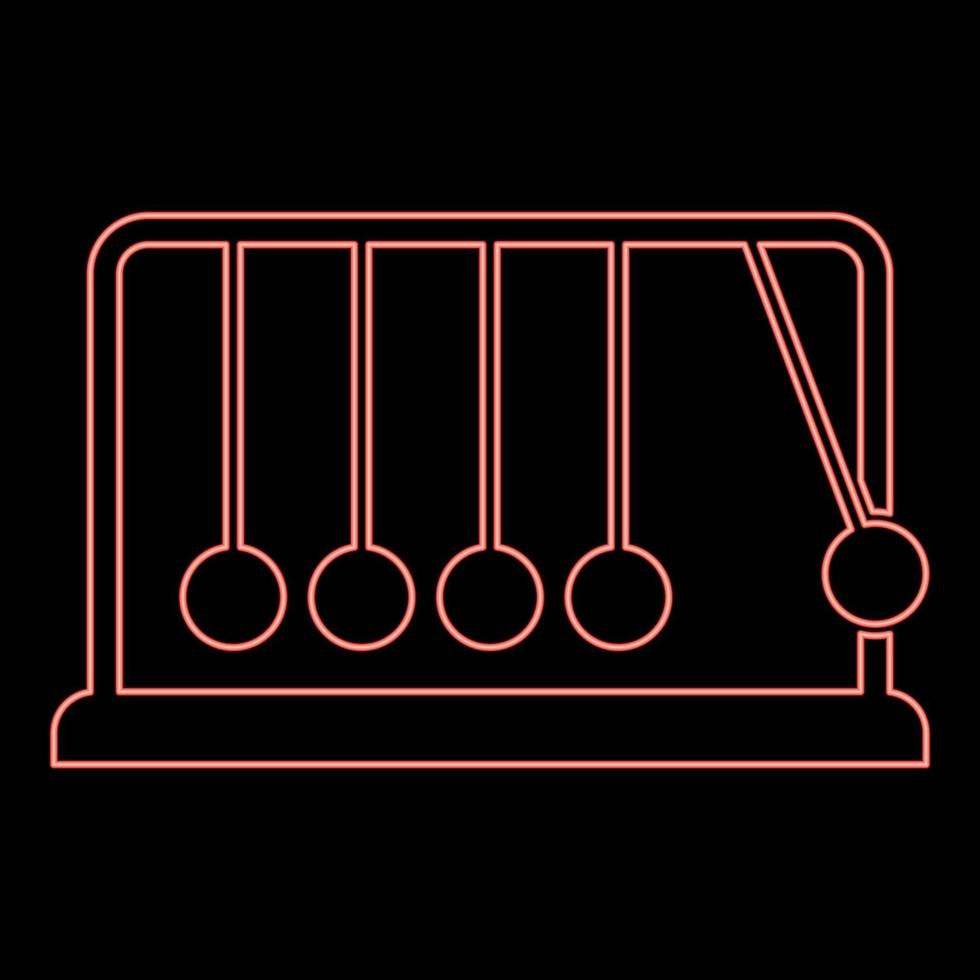This image is a minimalist graphic design of a Newton's cradle—a classic desk toy featuring five spherical balls hanging in a row by strings. The backdrop is a solid, deep black, which starkly contrasts with the delicate, reddish-orange to peach-pink lines that define the cradle and its components. Four of the balls hang vertically in a state of rest, while the fifth ball on the right is depicted as being pulled outward, ready to release and transfer its kinetic energy through the sequence of balls. The simplicity of the design is striking, with no additional elements to distract from the elegant depiction of the Newton's cradle.